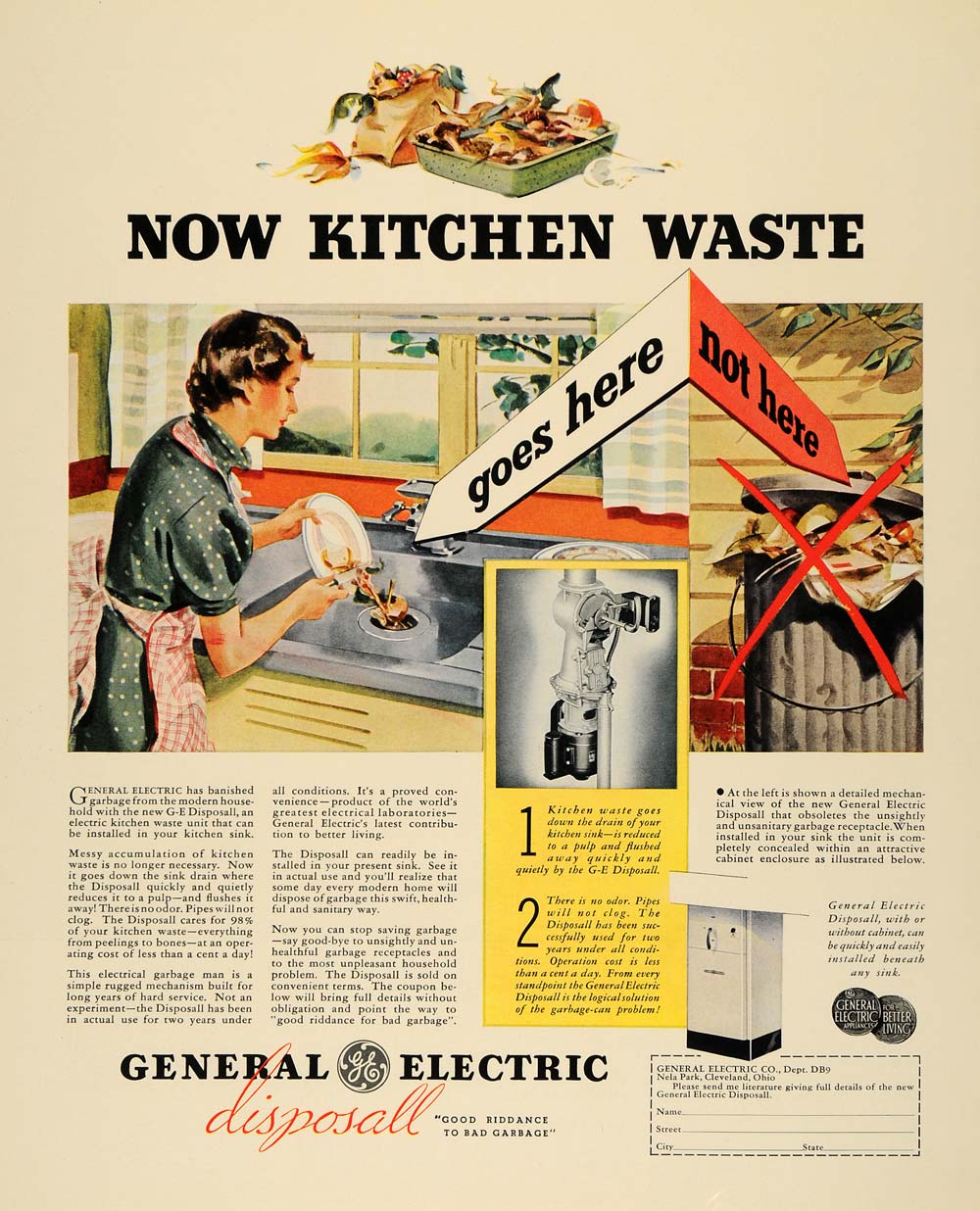The image appears to be an old magazine advertisement for a General Electric garbage disposal unit. The background is light brown, giving it a vintage feel. At the top of the page, there is a section with various food items, and it features the heading "Now kitchen waste goes here" with a white arrow pointing to a garbage disposal and "Not here" with a red arrow pointing to a garbage can with an 'X' over it. The main illustration depicts a woman at a sink, scraping food from a plate into the garbage disposal, contrasting sharply with the trash can image filled with waste. A black-and-white photograph in the middle of the page shows the inner workings of the disposal, accompanied by a yellow section that explains its operation in two steps. Below these images, the text explains the benefits and uses of the garbage disposal, with many paragraphs detailing the product. At the bottom of the page, there is a promotional tagline from General Electric: "Good riddance to bad garbage," followed by a call-to-action with a form for readers to request more information about the new General Electric disposal, complete with spaces for a name, street, city, and state.